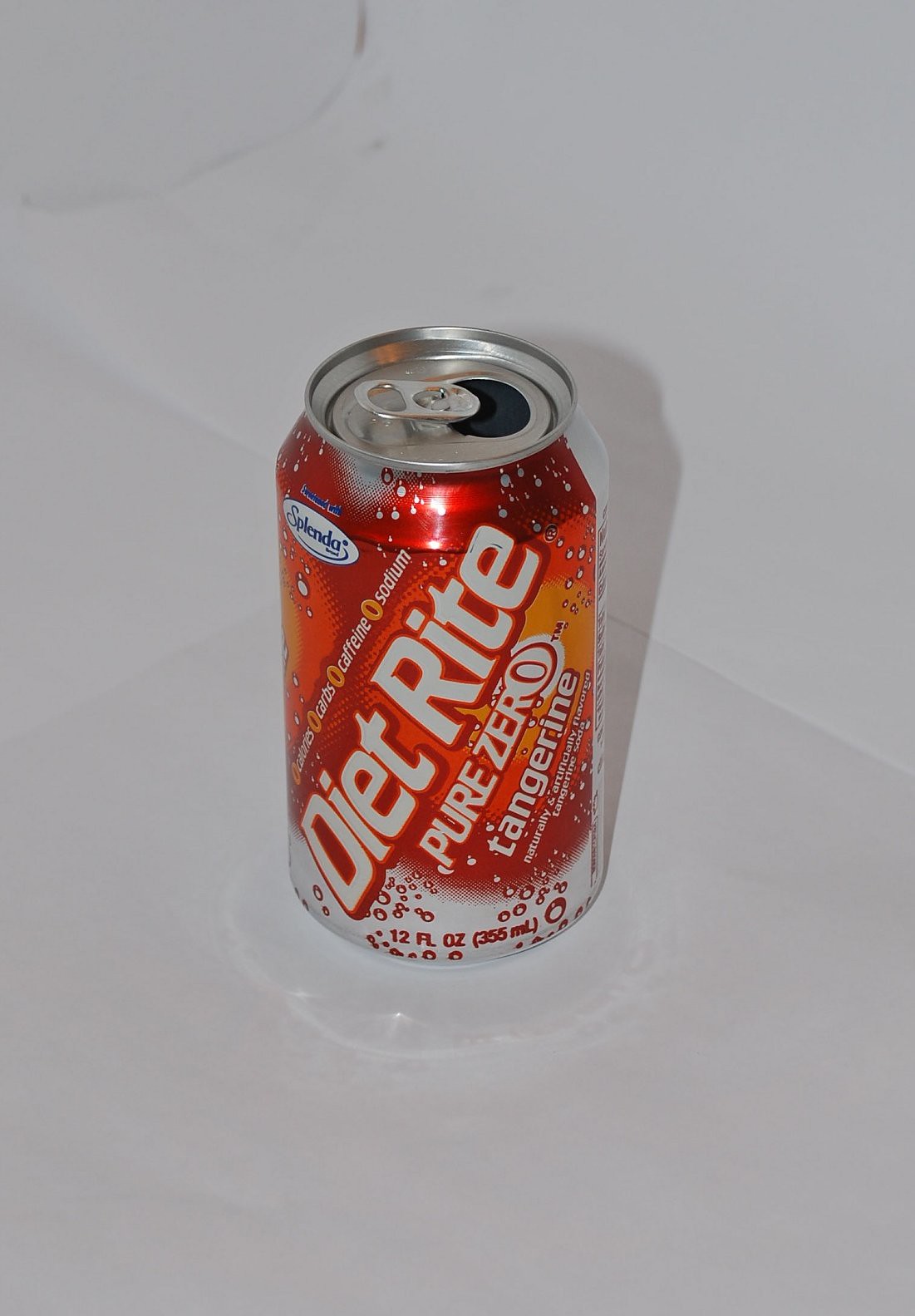This photograph captures a top-down view of an opened soda can set against a stark white background. The can features a silver top and a predominantly red body adorned with silver dots. Diagonally across the center, from the bottom left to the top right, the word "Dietrite" is prominently displayed in bold red-outlined letters. Directly below this, the phrase "Pure Zero" is written in white. Further down, in smaller white lowercase letters, the flavor "Tangerine" is indicated. Encircling the bottom edge of the can, a white strip bears red text. Additionally, on the upper left section of the can, a white oval label with "Splenda" inscribed in blue stands out, signifying the use of this sweetener.